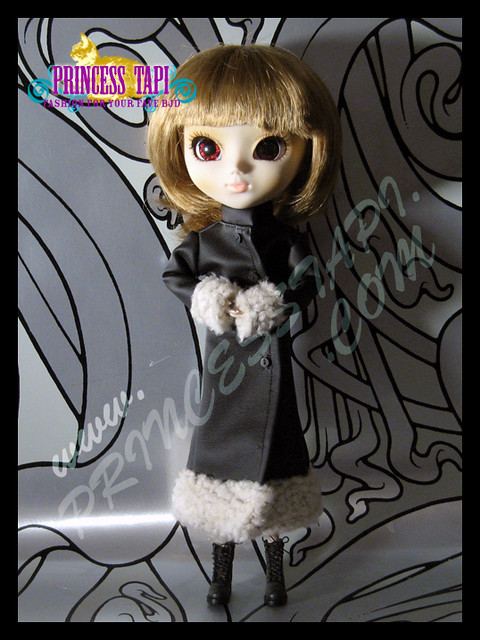The image depicts a striking and eerie doll with a large, pale head, sporting a bob haircut with dirty blonde or light brown hair and a blunt fringe. The doll's eyes are unusually large and reddish, with long lashes, adding to its unsettling appearance. It is dressed in a long, fashionable trench coat, black with white furry cuffs and hem, enhancing its chic yet haunting look. The background is a light gray with a detailed Paisley-like pattern, creating a subtle, textured backdrop that complements the scene. Towards the top left corner, there is an orange cat logo with purple text reading "Princess Tappy" and smaller pink text below that states "fashion for your favorite BJD." A watermark at the bottom reads www.princesstappy.com, indicating it might be an advertisement for the doll. The doll's outfit is completed with high-laced, brown or black combat boots, emphasizing its trendy yet eerie aesthetic.